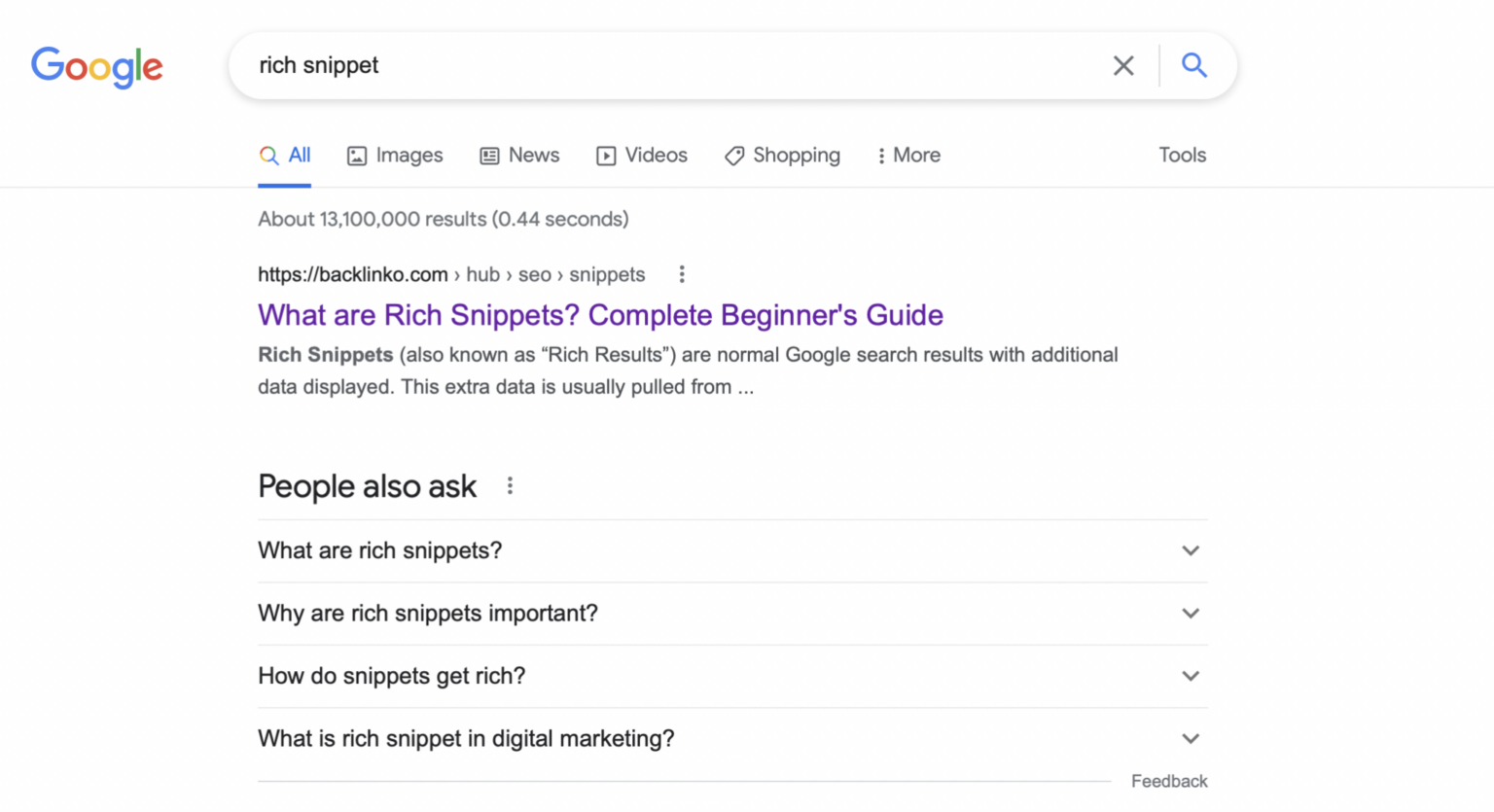Here is a more organized, detailed caption for the described screenshot:

---

Screenshot of a Google Search Results Page for “Rich Snippets”

In this image, we see the familiar layout of a Google search results page. Positioned on the right side of the screen is the iconic Google logo. Centered at the top, the Google search bar displays the query “rich snippet” within the text box.

Below the search bar are the category options: "All," "Images," "News," "Videos," "Shopping," "More," and the "Tools" option towards the far right. The search has returned approximately 13,100,000 results in a swift 0.44 seconds.

The first result displayed is a link to Backlinko’s page (https://backlinko.com) titled "What Are Rich Snippets? Complete Beginner's Guide." This result is listed as a hub for SEO snippets with a detailed description explaining that rich snippets, also known as rich results, are standard Google search results enhanced with additional data. The description snippet concludes with an ellipsis, indicating more information follows: “This extra data is usually pulled from...".

Underneath this result is the "People Also Ask" section, featuring related questions:
1. What are rich snippets?
2. Why are rich snippets important?
3. Why do snippets get rich?
4. Why so rich?
5. What are rich snippets in digital marketing?

This informative layout provides a comprehensive overview of rich snippets and their importance in the SEO landscape.

---